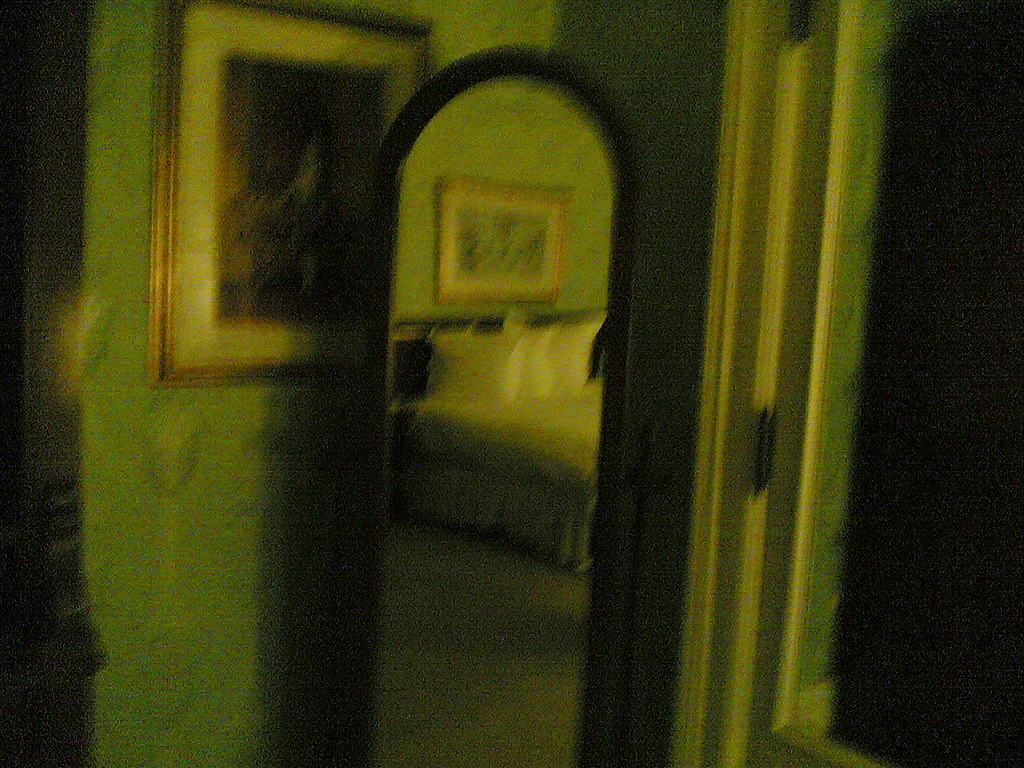This grainy and low-resolution image captures a somewhat eerie bedroom scene with a strong green tint permeating the entire picture. At the center, a dark-framed, floor-standing mirror reflects a portion of the room. The reflection reveals a bed adorned with red and green patterned bed coverings and three throw pillows. The bed's fabric extends down to the floor, resembling a dust cover. Above the bed hangs a framed picture, although its details are hard to discern.

The backdrop features two-toned green walls—lighter on top and darker paneling below—adding to the room's unsettling atmosphere. To the left of the mirror's reflection, there's another indistinct framed artwork, likely of a person, adjacent to a piece of dark furniture that might be an armoire. On the right side of the mirror, part of a white door frame or possibly a window with a curtain can be seen. Overall, the dark, greenish hue and grainy texture make it challenging to discern finer details, but the scene clearly captures the essence of a dimly lit, somewhat mysterious bedroom.